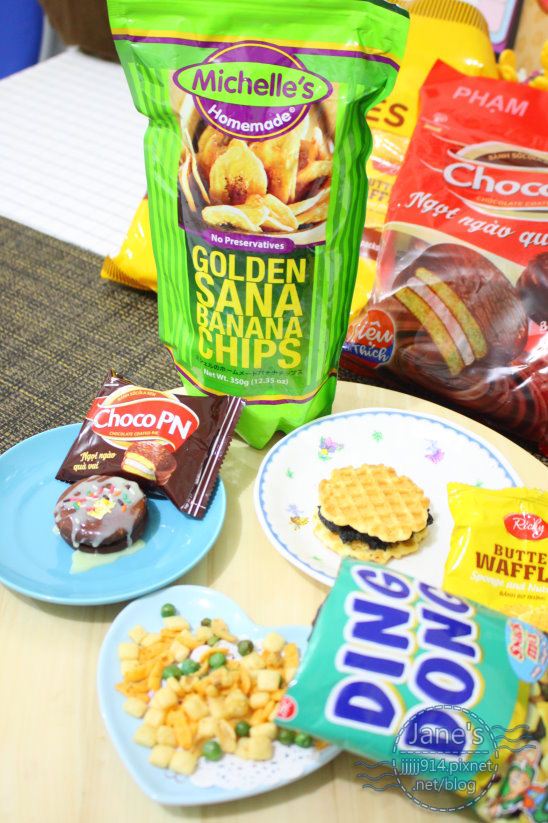This image captures a diverse array of snacks meticulously arranged on a table covered with a tablecloth. The setting appears to be indoors, probably a kitchen, though the time of day is indiscernible. On the left side of the table sits a blue plate with a chocolate biscuit topped with icing, labeled "ChocoPN". To the center bottom of the image, there is a bag of assorted crackers called "Ding Dong," with an appearance similar to Chex Mix. Above this, slightly to the right, a white plate holds a waffle sandwich, partially revealing yellow packaging labeled "buttermilk waffle." On the bottom right corner of the image, several bags of snacks are visible, including "Michelle's Homemade Golden Sana Banana Chips" in a tall green bag, accompanied by other snack bags written in different languages. The colors in the image include tan, blue, brown, black, red, yellow, green, light blue, dark blue, orange, and lime green, giving it a vibrant appearance. The objects are well spaced, and no single item dominantly occupies the center of the image.